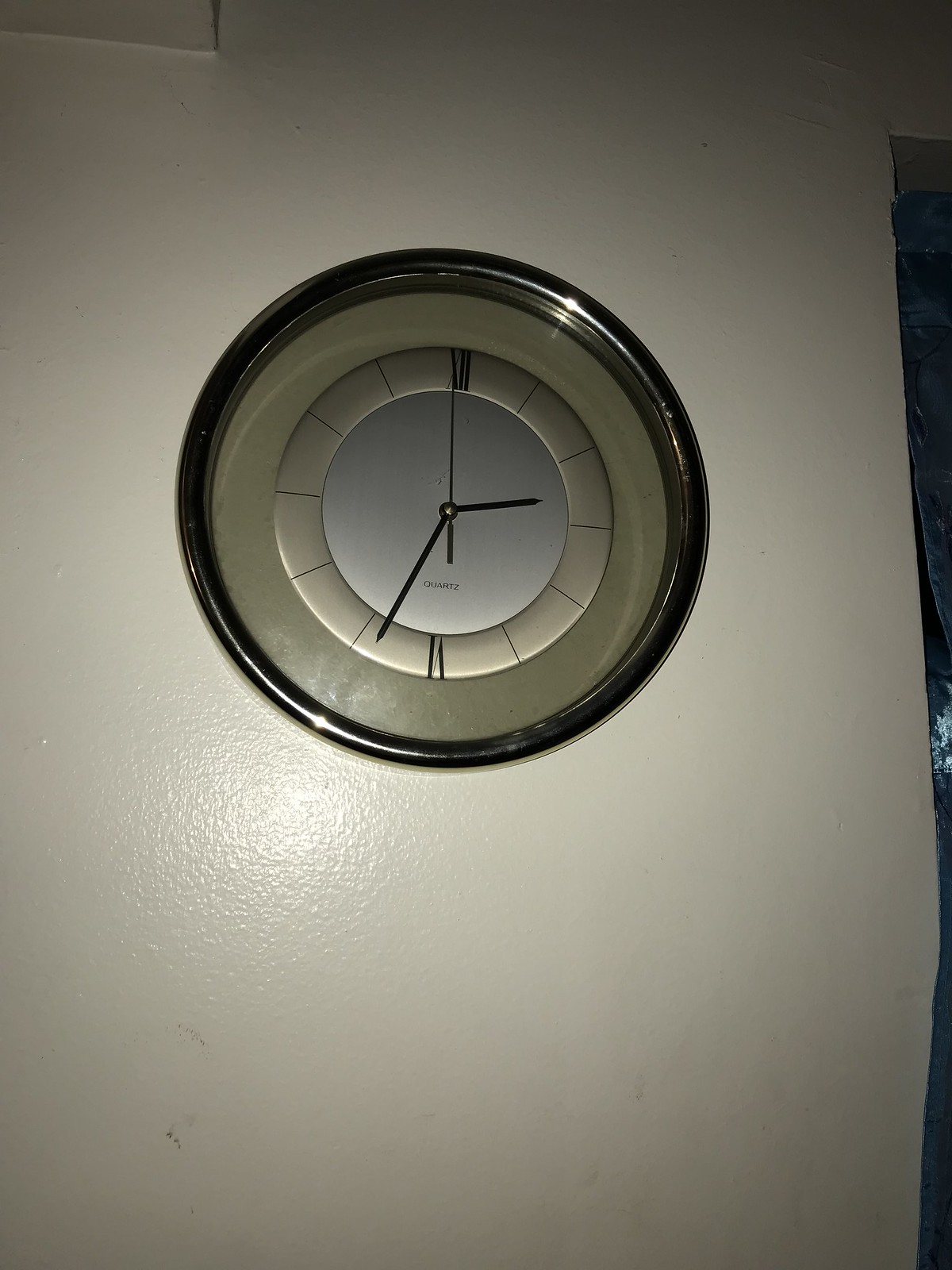This image features a clock mounted on a white or cream-colored wall. The clock's design is both sleek and modern, with a polished black rim encircling its perimeter. Inside this black border is a second, slimmer silver border, followed by yet another concentric silver ring, giving the clock a layered look. The clock's face, showing the time as 2:34, is clean and minimalistic. The black hands are thin and sharply contrast against the light background. Instead of traditional numerals, the clock features simple black lines to mark the hours, creating an impression of elegance and simplicity. The overall aesthetic is refined, combining functional design with understated sophistication.